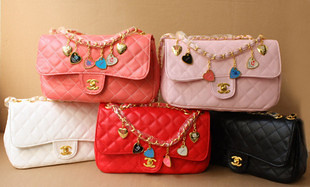This photograph showcases five leather Chanel handbags arranged against a tan cream-colored backdrop. Each handbag, exhibiting a quilted diamond pattern on its leather facade, is adorned with intricate attachments and metallic embellishments. The ensemble is presented in two rows; the top row features a vibrant hot pink handbag on the left, which is accented with blue, black, and white charms, while the lighter pink handbag on the right is decorated with similar colored attachments. On the bottom row, the white handbag to the left shines with a gold Chanel insignia, symbolized by the interlocking C's in a metallic brass or gold finish. The middle bag is striking in red, adorned with green, blue, and pink elements hanging from a chain. Completing the bottom row, the black handbag on the right mirrors the white one with its iconic gold insignia. Each bag, reflecting Chanel's classic elegance and sophisticated design, suggests this image is either a display for a collector's showcase or a high-end listing, possibly for sale on a platform like eBay.